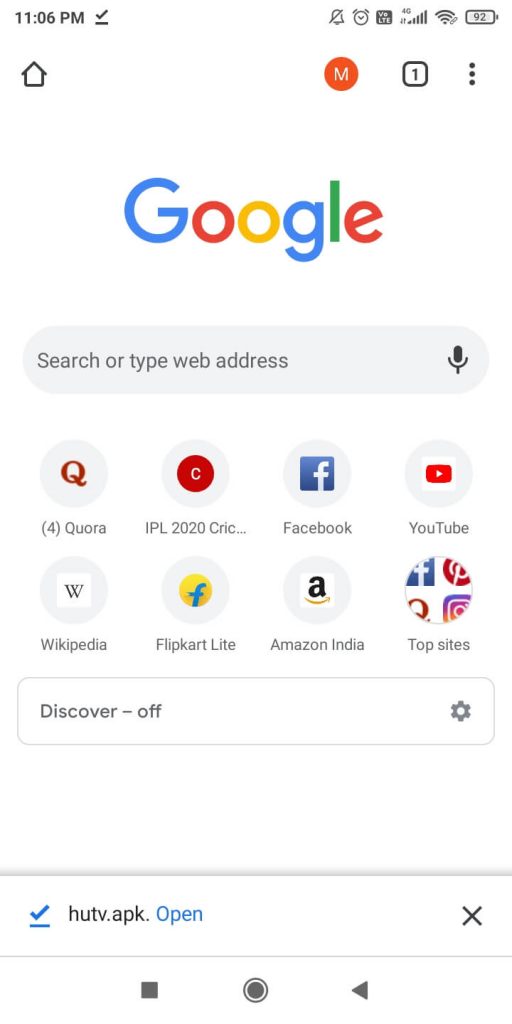The screenshot, taken from a cell phone at 11:06 PM, showcases various elements on the screen. A checkmark appears next to the time, indicating possibly a notification or a network status. The battery is at 92%, accompanied by a battery icon, along with a Wi-Fi symbol and the text "LG LTE". The Google logo appears in its classic blue, red, yellow, and green colors. Below the search bar, which prompts "Search or type web address" and includes a small microphone icon for voice input, a series of app icons are displayed.

Prominently, the Quora icon, characterized by its red and grey color scheme, and a text labeled "IPL 2020" are visible. Also present are a circle icon with a letter "C", the blue and white Facebook logo, and the YouTube logo featuring a red and white play button. Additionally, there are icons for Wikipedia, Flipkart Lite, and Amazon India, denoted with the Amazon logo and a small "a".

Under these icons, the text "Top Sites" is displayed, followed by "Discover / Off". Beneath this section, there is a clickable blue text labeled "HUTV.APK.open".